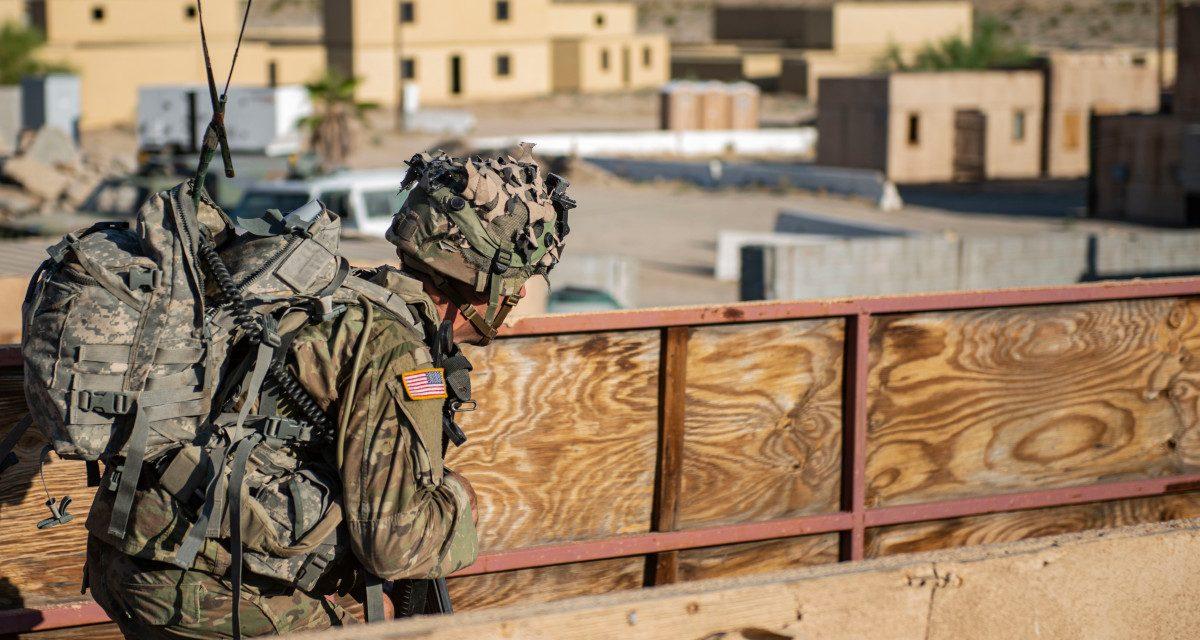In the image, we see a military scene taking place during the day in what appears to be a warmer climate, possibly indicating a non-Western country. Dominating the foreground on the left is an American soldier clad in camouflage fatigues, complete with a helmet and an American flag patch sewn onto his right shoulder. He is partially ducked behind a wooden structure, possibly a bridge or fence, suggesting he is taking cover. The soldier is heavily equipped, with straps and wires visible over his uniform and a large, overstuffed backpack on his back, indicating he is carrying a significant load of supplies. Only visible from the hips up, he appears to be leading or part of a convoy, hinted at by the shadow of another person behind him. In the background are several rather nondescript beige buildings, each featuring doors and two rectangular windows, reinforcing the military facility setting. The out-of-focus backdrop and the soldier’s cautious posture convey a sense of tension, hinting at the potential for imminent conflict.